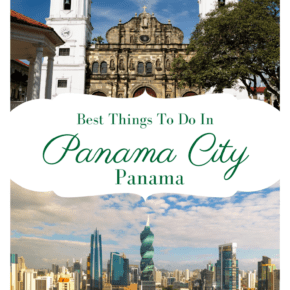A stunning panoramic view of Panama City showcasing a mix of architectural styles at sunset. In the center, a historic church with two distinct towers stands out, with one tower on the left and another on the right. Above, a white star appears against a brilliant blue sky, dotted with fluffy white clouds. The skyline features a variety of tightly-packed urban buildings, including a prominent spiral skyscraper. Green text on the image reads, "Best things to do in Panama City, Panama." The image perfectly captures the contrast of sunlight illuminating the left side of the city, while the right side remains in shadow.